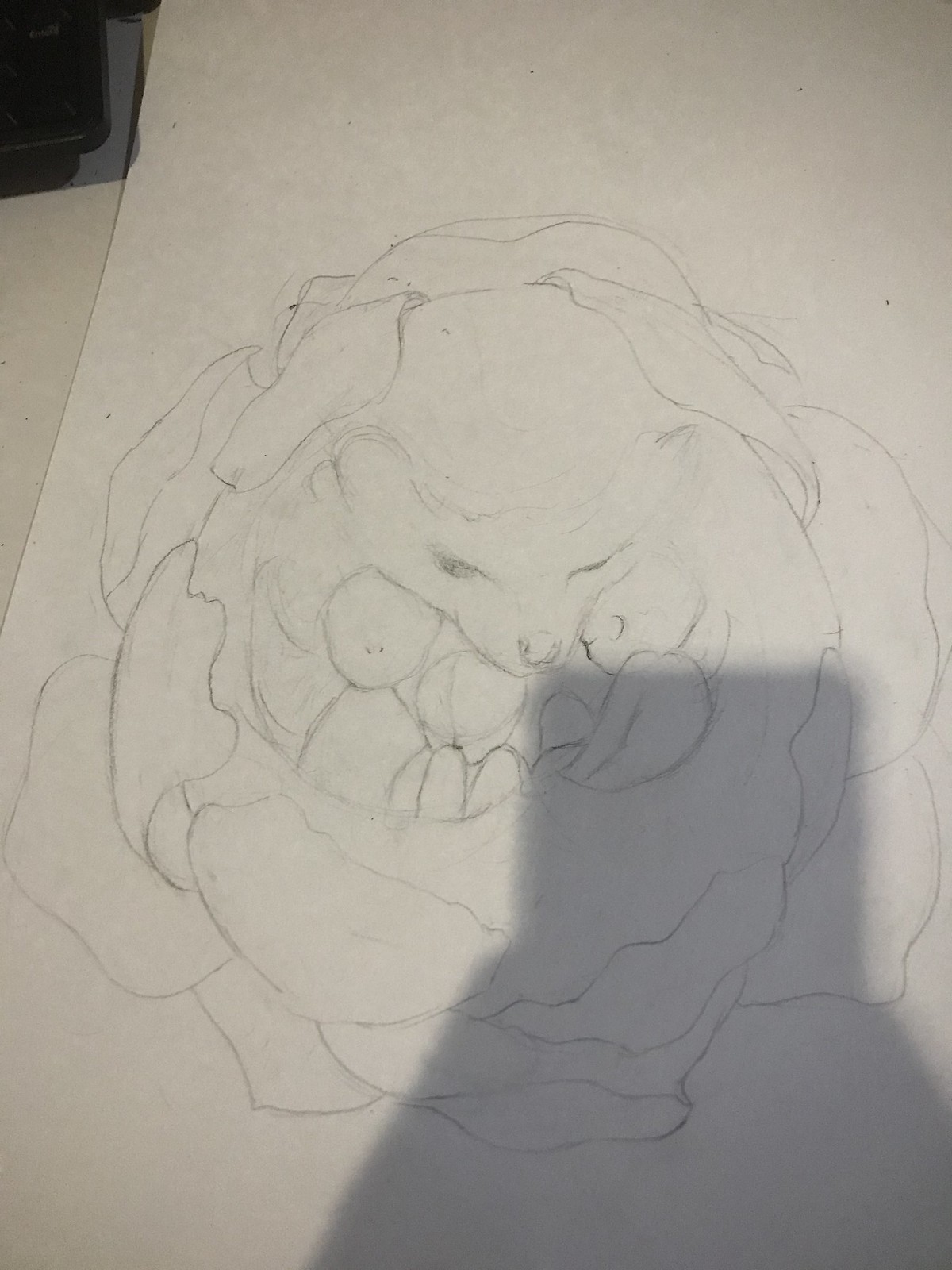This detailed black and white pencil sketch, drawn on cream paper, depicts a unique, armored creature resembling a hedgehog curled up in its defensive ball shape. Instead of spikes, the creature's back is covered in circular plates, reminiscent of pleated armor. At the center of this protective formation, three small children are warmly embraced by the creature. This intricate drawing also invokes the idea of inner seeds of a flower, with surrounding petal-like structures providing additional layers of protection. Captured in portrait mode, the photograph of the sketch includes the faint shadows of the artist's hands and their cell phone in the lower right-hand corner, adding a personal touch to this beautiful and evocative piece.